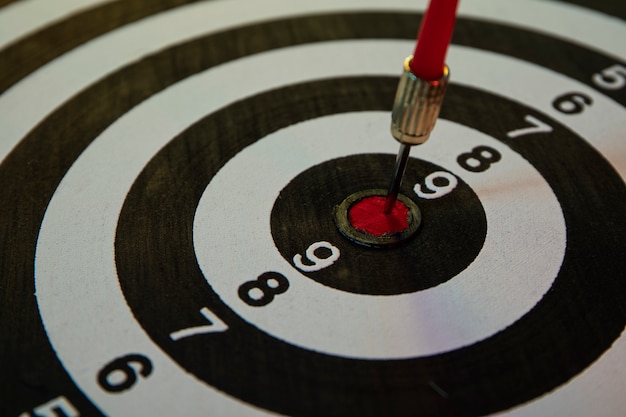The image is a close-up shot of a bullseye target with black and white concentric circles. At the very center is a red dot, indicating the bullseye, which has a red dart precisely embedded in it. The dart features a black end leading into a silvery, chrome-like body, and its neck appears to be red. Surrounding the red center, the target displays numbers in a sequence, starting from 9 next to the bullseye, followed by 8, 7, 6, and 5, both above and below, denoting the point values of each ring. The alternating black and white circles create a stark contrast, highlighting the scoring sections that taper off as they extend outward from the middle.